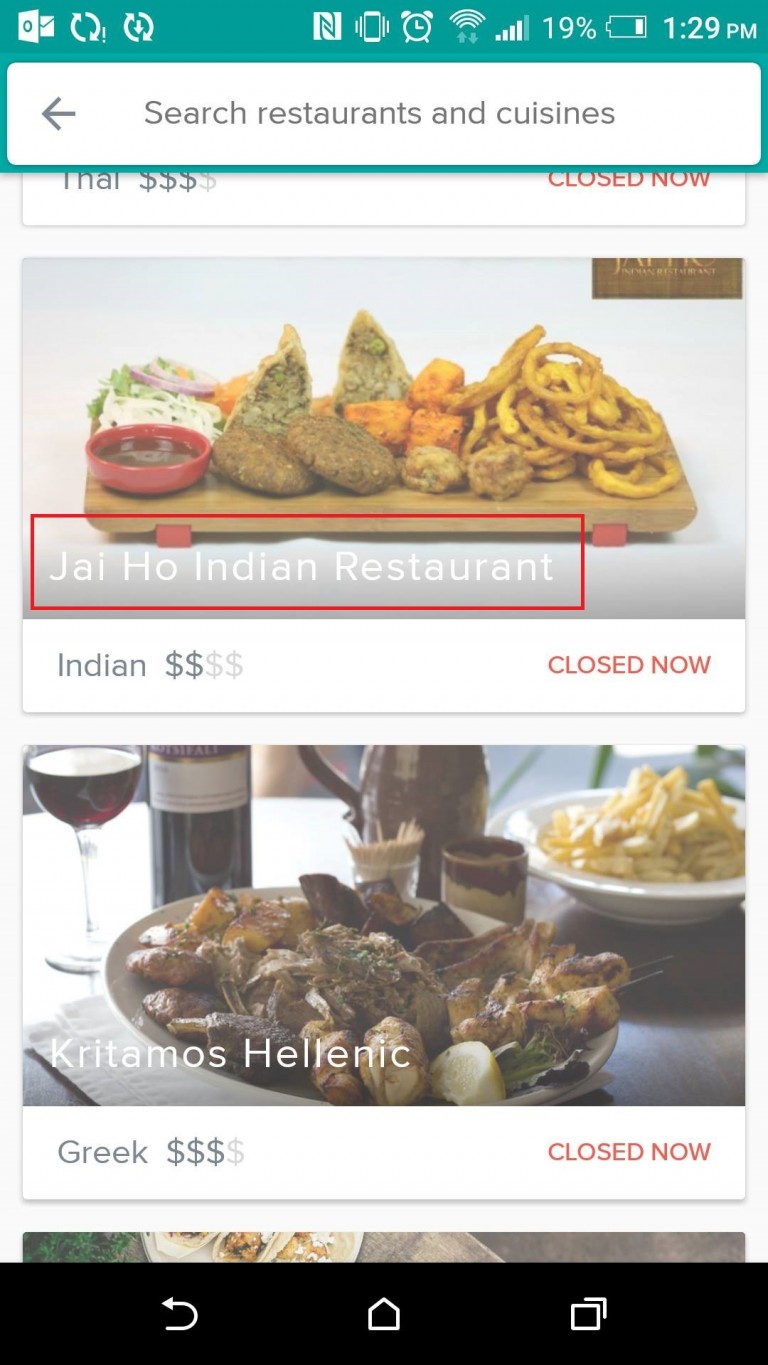In this image, we are presented with an online restaurant and cuisine search page viewed on a mobile device. The search bar at the top, displaying the text "search restaurants and cuisines" in small, black letters, confirms the functionality of the page. The top-right corner provides current time and phone status details: it's 1:29 PM, the battery is at 19%, and the signal strength is robust with four out of five bars highlighted. Additional icons indicate that the phone is on vibrate and there's an unread mail notification on the left-hand corner.

Further down the page, we see a list of two restaurant options. The first image features a vibrant, rectangular photo showcasing an assortment of Indian cuisine, including appetizing samosas and other snacks accompanied by dipping sauces, from "Jai Ho Indian Restaurant." Despite its appealing offerings, the restaurant is currently closed. Its pricing is moderate, with two out of four dollar signs filled.

Beneath it is another restaurant, "Krytomos Helenik," specializing in Greek cuisine, as indicated by the label beneath its name. This establishment, noted for its more upscale pricing with three out of four dollar signs filled, is also closed at the moment. The image associated with this listing exudes elegance, featuring a wine bottle and glass alongside a plated Greek dish. The meal includes meat, a lemon wedge, and what appears to be chips or similar items in a bowl, all presented in a visually appealing manner.